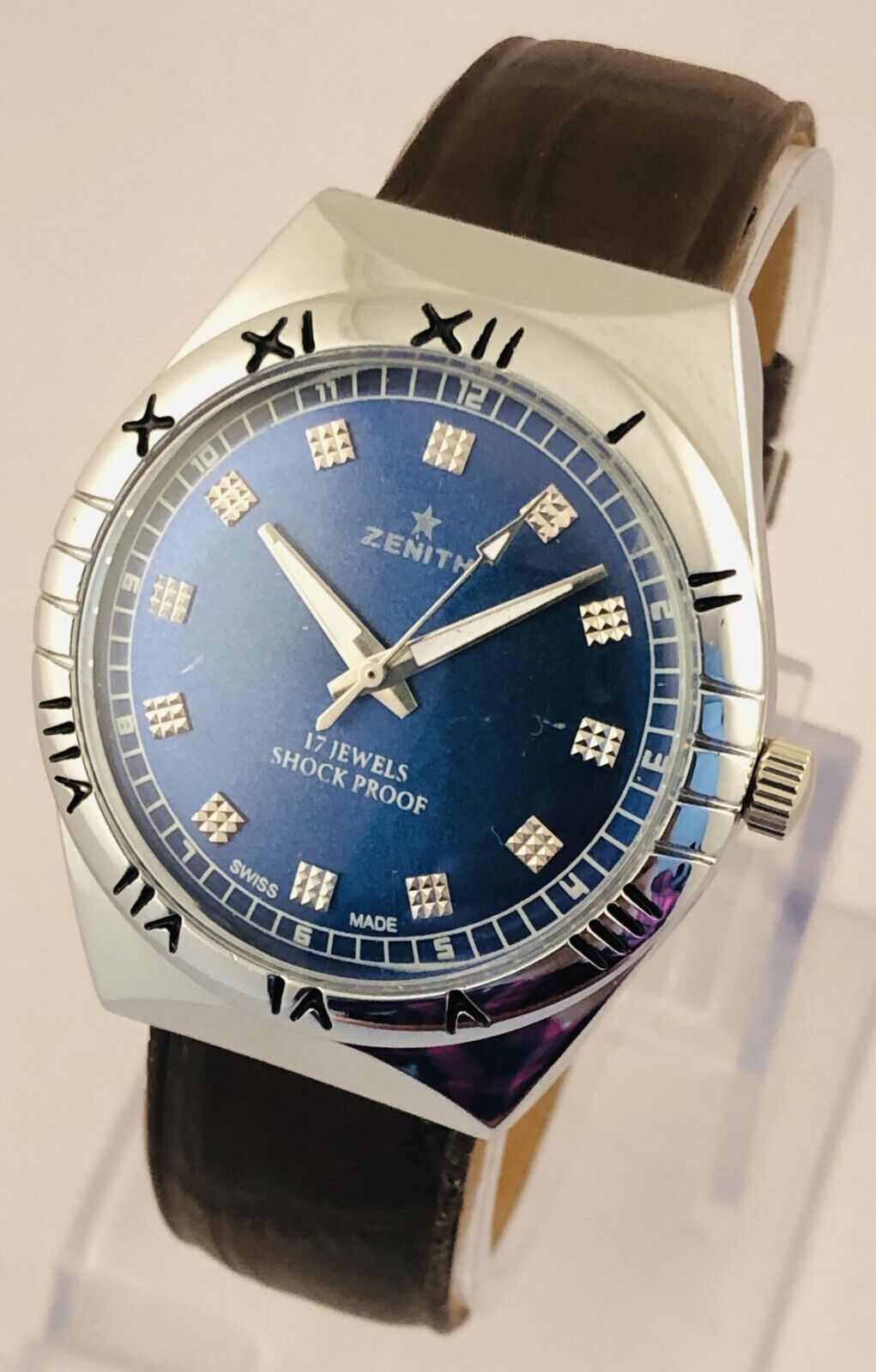This close-up indoor photograph captures an elegant wristwatch placed on an acrylic stand. The timepiece features a brown, texturized leather wristband paired with a silver frame. The watch face is a deep navy blue, adorned with silver-colored Roman numerals from 1 to 12, with additional jewel-like decorations at each hour mark, except for 3 and 9. Central on the dial is the brand name "Zenith" with a star emblem above it, and the inscriptions "17 Jewels," "Shockproof," and "Swiss Made" below the hands.